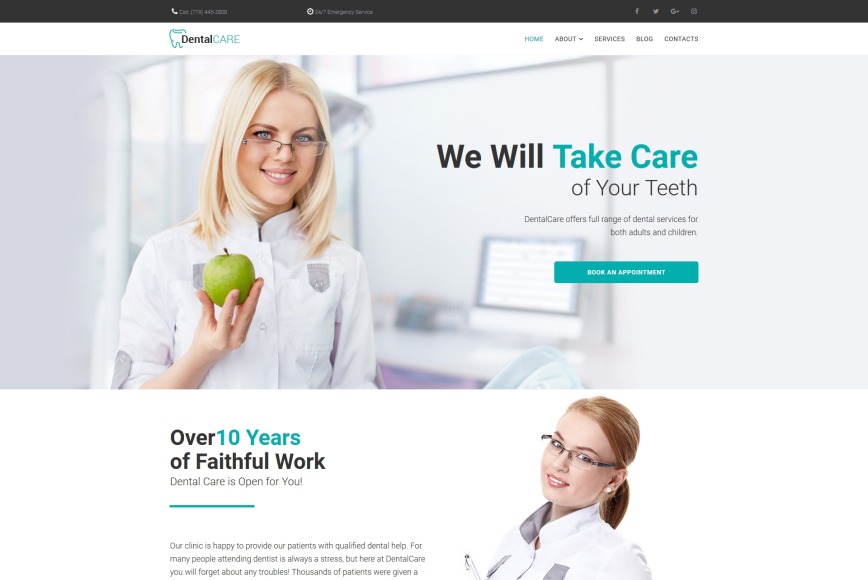A screenshot taken from a dental website features a black navigation bar at the top, which contains several elements on the right side. Although the text is not entirely legible, it includes a phone number formatted in white font that is not clearly identifiable as a toll-free 1-800 number. Adjacent to the phone number are icons resembling a gear or possibly a clock, followed by social media logos for Facebook, Twitter, and Google Plus, suggesting the screenshot may be somewhat dated. Further to the right, there's an icon that appears to represent a printer.

On a white background below the navigation bar, there is a grey tooth icon accompanied by text: the word "dental" in black and the word "care" in blue. To the right of this logo, the menu items "Home," "About," "Services," "Blog," and "Contact" are listed in black text.

The main section of the webpage features a stock photo of a blonde woman wearing glasses and a bluish shirt, standing in an office environment with a computer in the background. She is holding a green apple in her left hand. Overlaying this image are the words: "We will" in black text, "take care" in green text, and underneath, "of your teeth" in black text.

Below this section, there is a call-to-action button labeled "Book an Appointment." Near the bottom of the screenshot, another generic image shows a woman dressed in a dental cleaning uniform, attempting to appear stylish. She has glasses and blonde-tinted hair, although she seems different from the woman in the previous image. The accompanying text highlights the dental practice's ten faithful years of service.